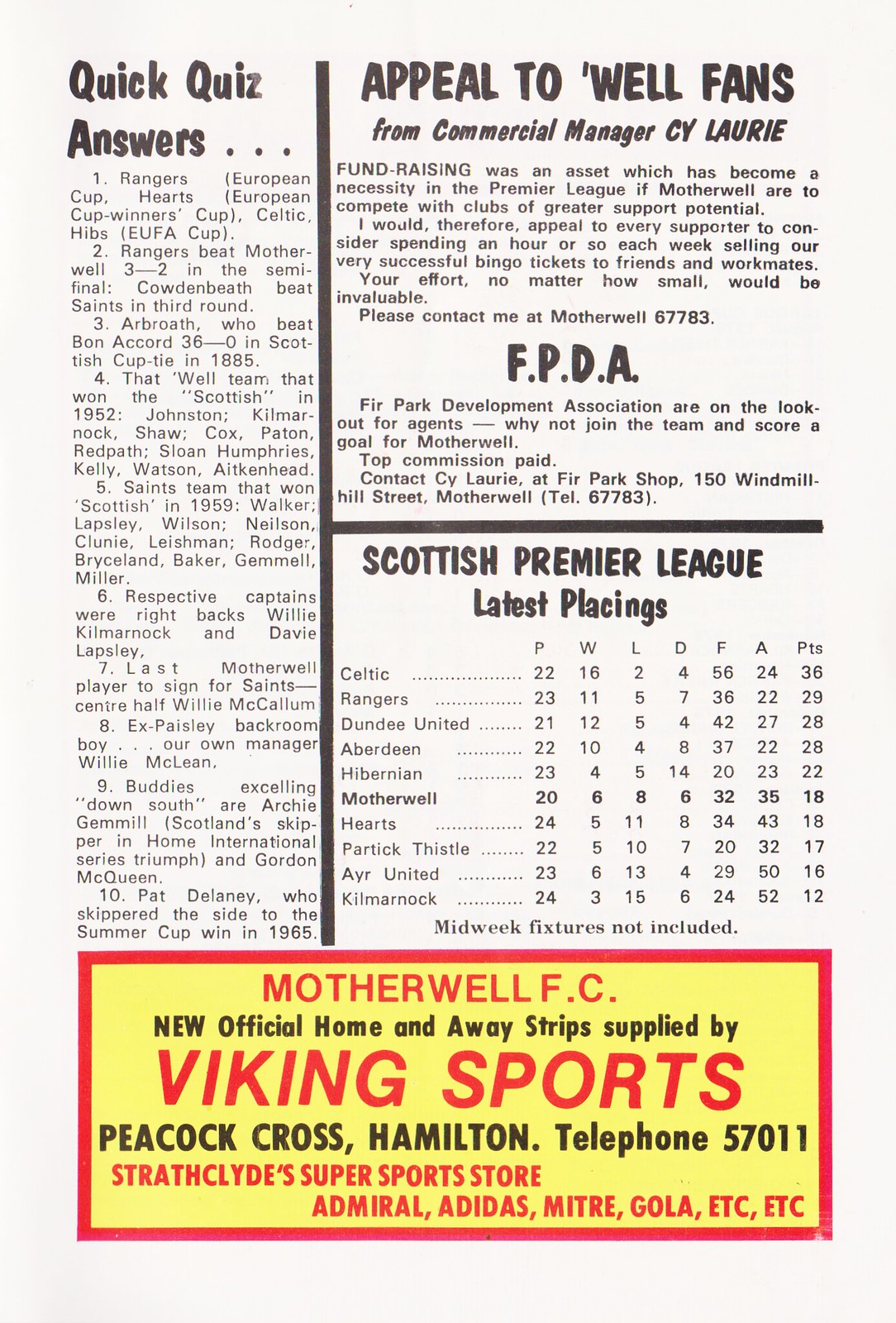The image appears to be an old game day program page from the Scottish Premier League, reminiscent of the 1950s or 60s based on the design and colors. Predominantly black and white, the bottom quarter of the page features a vibrant yellow background with a red border and red lettering. The advertisement in this section promotes "Motherwell FC" with a headline stating, "New official home and away strips supplied by Viking Sports," followed by the contact address, "Peacock Cross Hamilton, telephone 57011," and the tagline, "Strathclyde's Super Sports Store, offering brands like Admiral, Adidas, Mitre, and Gola."

On the left side of the page, an upper column titled "Quick Quiz Answers" provides information in black lettering. Adjacent to it is a heading, "Appeal to Well Fans," where commercial manager Cy Lowry encourages supporters to participate in fundraising by selling bingo tickets, emphasizing the importance of such efforts for the club’s competitiveness in the Premier League. 

Centrally placed is a table labeled "Scottish Premier League Latest Placings," listing teams like Celtic, Rangers, and Dundee United along with their win-loss records and points. The text surrounding the table offers additional game-related data and commentary, providing a comprehensive snapshot of the league standings and scores. Overall, the page effectively blends historical sports reporting with contemporary promotional content.